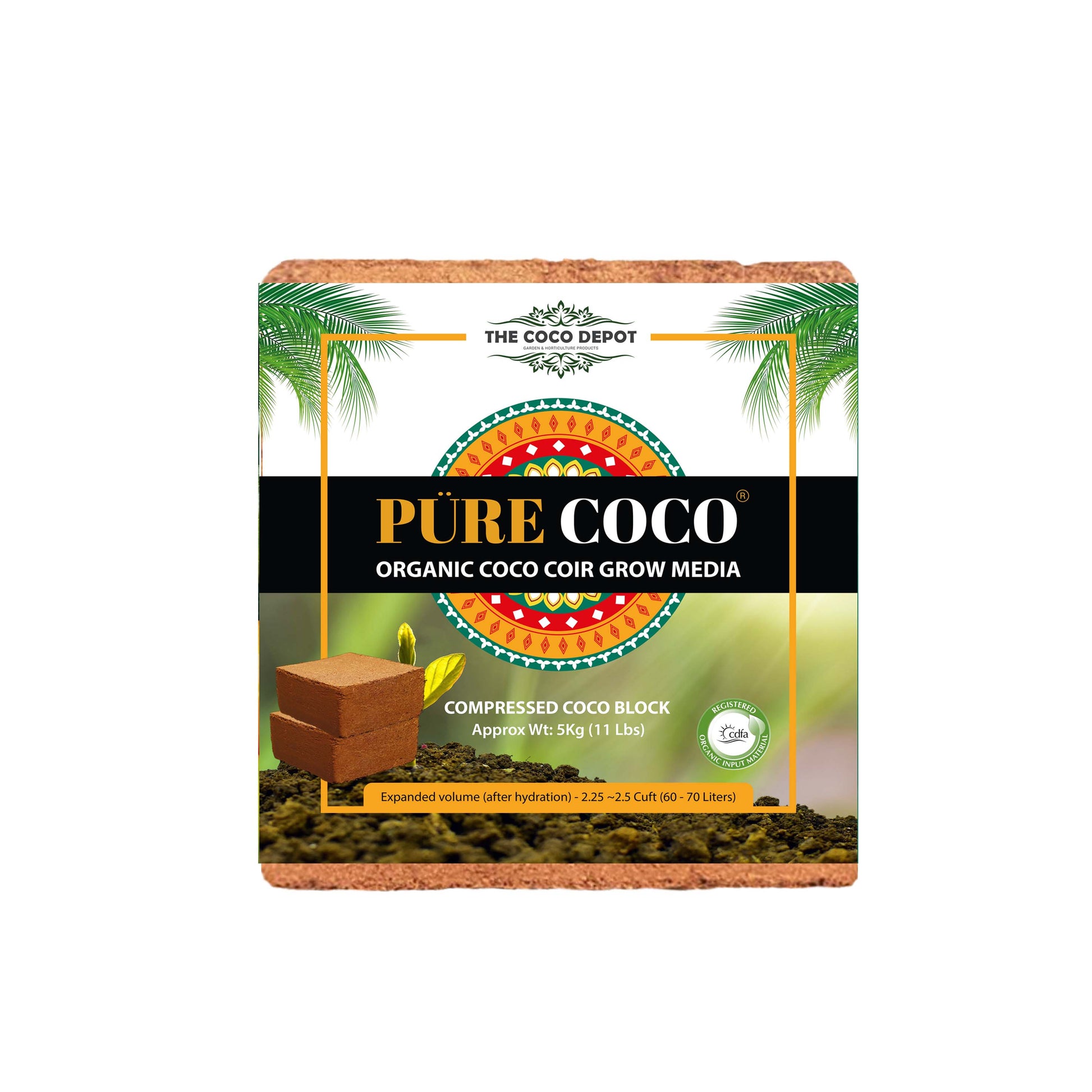The image is an advertisement for a product from the brand "Cocoa Depot." The label prominently features the text "Pure Cocoa, Organic Cocoa COIR Grow Media," stating that it contains "Compressed Cocoa Block." The top of the image showcases the "Cocoa Depot" logo against a white background accented with two palm tree fronds. 

The packaging details expanded volume post-hydration as 60 to 70 liters, and a weight of approximately 5 kilograms or 11 pounds. To the left of the label, there is a small image depicting two cocoa blocks, while the lower right bears a green logo or seal, though its text is unclear. 

The label itself is set against a backdrop with a mix of natural textures, such as palm fronds and dirt. Toward the lower section, a distinct black title box features the product name, with "Pure" highlighted in orange-yellow lettering matching the surrounding yellow square. The circle within this yellow square features an array of colorful patterns, including diamonds, squares, and triangles in green, white, orange, yellow, and red.